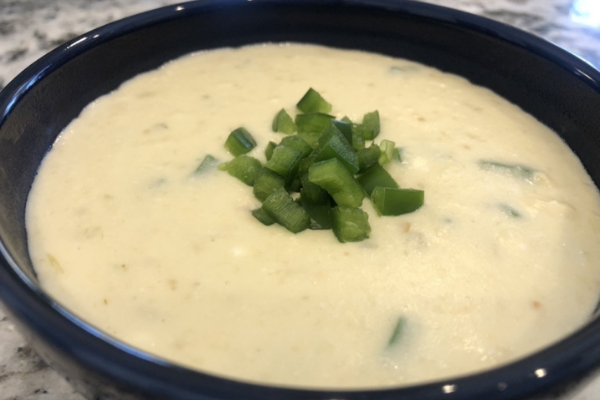The photograph captures a close-up of a large black bowl, occupying nearly the entire frame, set on a whitish-black marble tabletop. The bowl contains what appears to be a thick, creamy soup with an off-white or light creamy color, reminiscent of cream of mushroom or chowder. At the center of the bowl, there is a prominent pile of chopped green bell peppers or scallions, which stand out vividly against the soup's pale background. Additional bits of green peppers and possibly other vegetables are dispersed throughout the soup, adding texture and color to the dish. The light source, coming from the upper right, creates a slight glare on the bowl, emphasizing the indoor setting of the photograph.